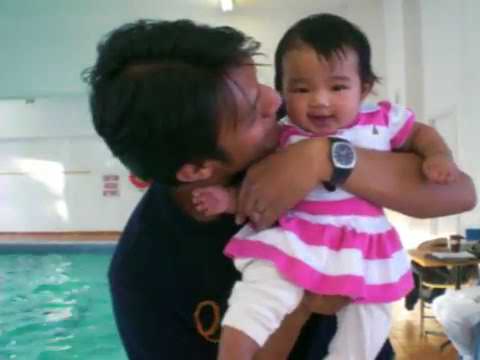In this square digital photograph, a man with straight black hair and brown skin is seen holding his 9-10 month old baby girl at an indoor swimming pool. The background features white walls and ceiling with greenish-blue water in the pool. Some brown flooring and a table with a coffee cup and chairs are visible to the right. The man, dressed in a blue shirt, has his left arm wrapped around the baby, supporting her from underneath. His left wrist, adorned with a black watch, is prominently visible as he holds her close, their faces nearly touching as if he’s about to kiss her. The baby girl, possibly of Asian descent, with short straight black hair, smiles directly at the camera. She’s wearing a pink and white striped dress paired with white leggings. The image captures a tender moment of interaction and joy between the father and his daughter.